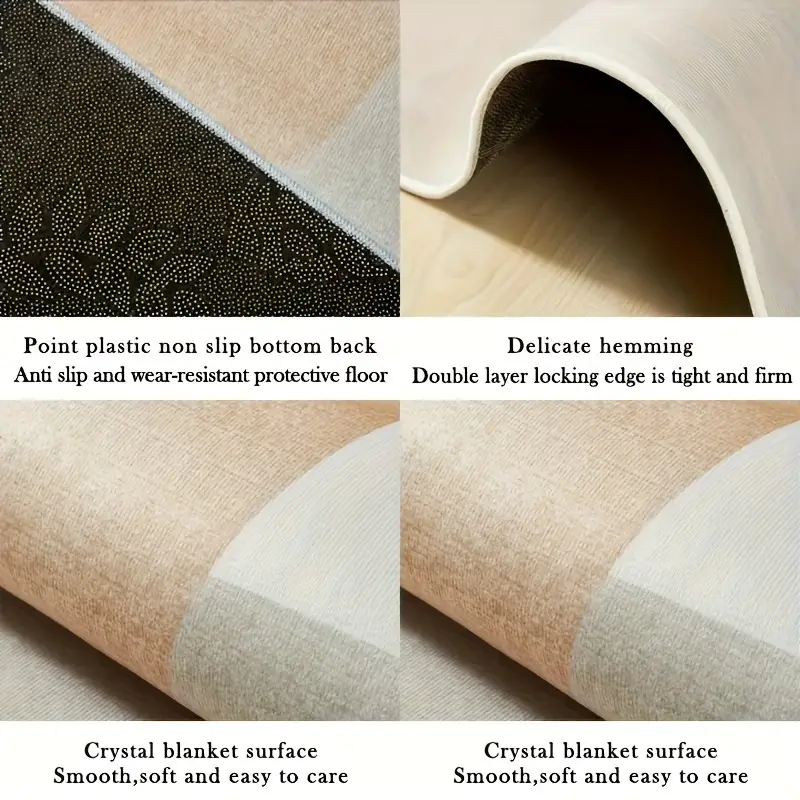The image is a square screenshot from a product description page divided into four evenly spaced panels, each showcasing different features of a non-slip mat or rug. The first panel, located in the upper left corner, displays the back side of the rug and features text that describes it as having a "point plastic non-slip bottom back," emphasizing its anti-slip and wear-resistant properties, suitable for protecting floors. Adjacent to this, the second panel features a close-up of the rug's edge, highlighting "delicate hemming, double layer locking edge," which is described as tight and firm. The third panel focuses on the surface texture, labeled as a "crystal blanket surface," noted for being smooth, soft, and easy to care for. The fourth panel redundantly restates the information about the crystal blanket surface. This cohesive visual presentation underscores the rug's durable backing, sturdy edges, and comfortable, manageable surface, making it clear this product is designed for effective, long-lasting floor protection.